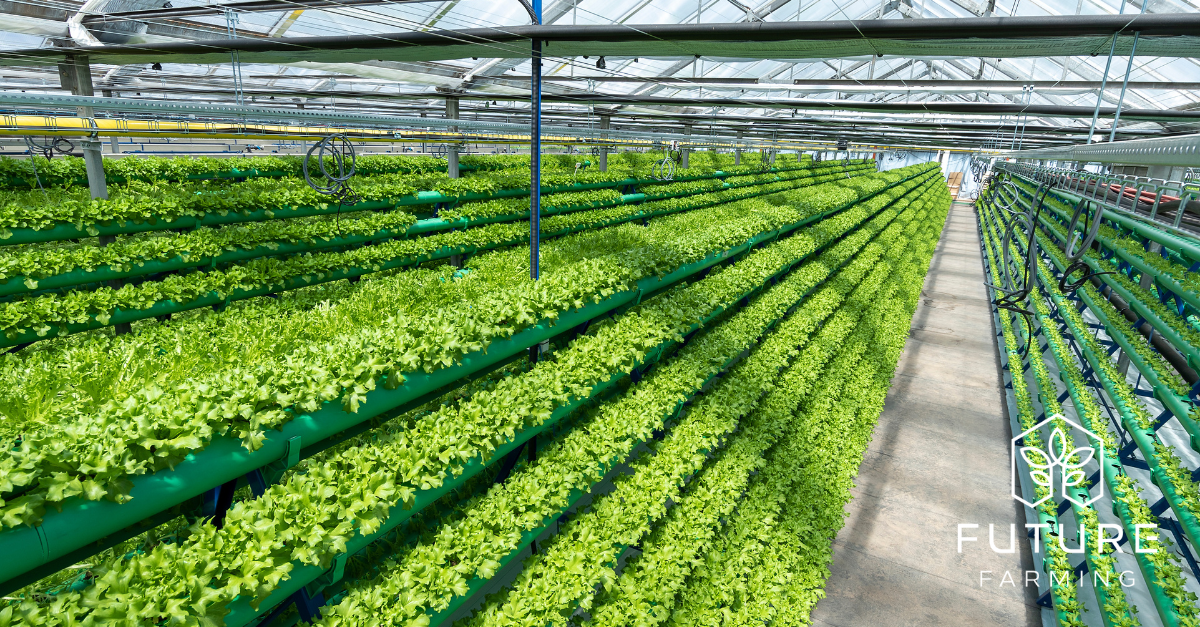The photograph depicts an expansive interior view of a greenhouse or growing room, showcasing a state-of-the-art, future-oriented farming operation. The image captures a high-angle perspective inside the building, allowing a comprehensive look at the setup. There are four separate lines of growing platforms extending from the foreground to the background, each fitted with six to seven distinct growing areas. These stands are densely packed with vibrant green plants, possibly vegetables or leafy greens, in various stages of growth.

To the right of the image, a packed dirt pathway is visible, stretching the entire length of the greenhouse. Above the rows of plants, robust irrigation systems are in place, spanning the entire area from the front to the back, ensuring even watering across all plants. The ceiling features an open glass roof allowing natural sunlight to pour in, enhancing the midday light that bathes the greenhouse in a warm, inviting glow.

On the far right, slimmer and tinier shelves also hold plants, creating a sense of depth and variation in the arrangement. There is no human presence in the photo, emphasizing the advanced and automated nature of this farming concept. In the lower right corner of the image, a logo depicting a plant and the text "Future Farming" is prominently displayed, reinforcing the innovative and forward-thinking theme of this agricultural setting.